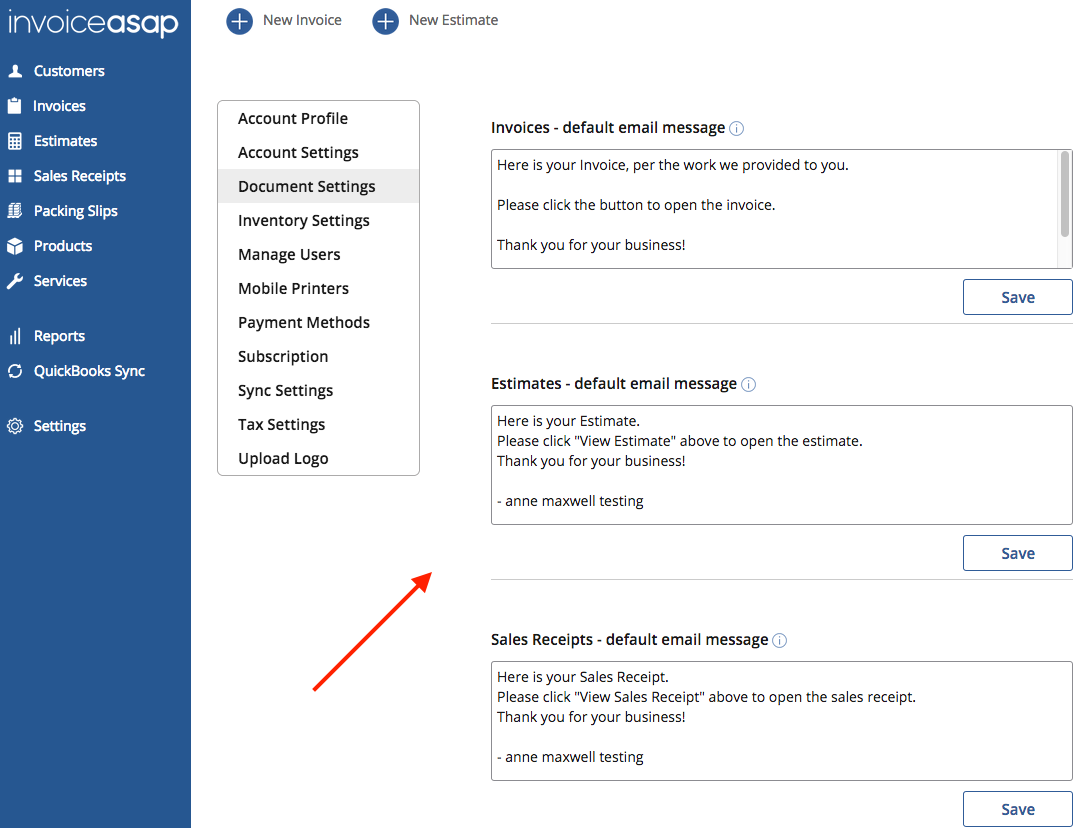This is a screenshot of specialized invoice software. The interface features a blue vertical navigation bar on the left, prominently branded as "Invoice ASAP" at the top. Below this, the menu includes key functional areas such as Customers, Invoices, Estimates, Sales Receipts, Packing Slips, Products, Services, Reports, QuickBooks, Sync, and Settings. The main white viewing pane on the right is divided into submenus for Account Profile, Account Settings, and Document Settings. Adjacent to this are options for configuring Invoices, Default Email Message, Estimates, Default Email Message, and Sales Receipts, Default Email Message. The screenshot likely illustrates the setup process for creating an invoicing and billing system tailored to company needs.